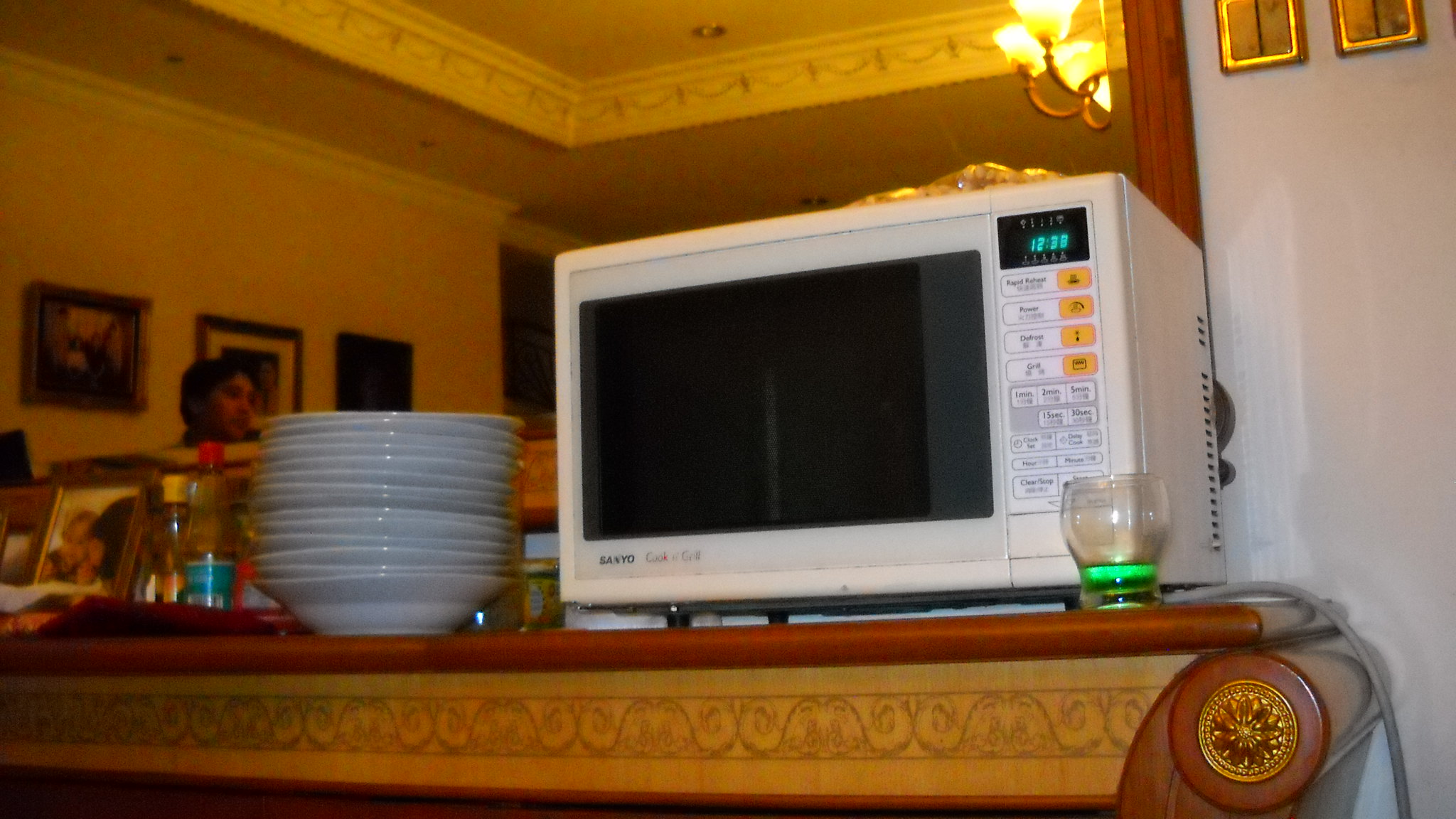This detailed image depicts a white microwave with orange and white buttons and a green display reading 12 o'clock, positioned on an ornate mantle or long table. In front of the microwave, to the right, is a small, rounded glass. To the left of the microwave is a stack of white bowls, with a couple of bottles of hot sauce nearby and possibly a bottle of soy sauce. On the far left of the mantle, a framed photo is visible. 

A large mirror behind the microwave reflects the rest of the room, showing three framed prints on the left wall, white crown molding, and ceiling molding in a cut-out section of the ceiling. A partial view of a chandelier is also visible on the right side of the mirror's reflection. The area appears to be a dining room or a restaurant-like setting, with a person partially visible in the mirrored background, suggesting it might be a staff or pickup area. The space is decorative with etched designs and a gold round motif on the sides of the mantle.